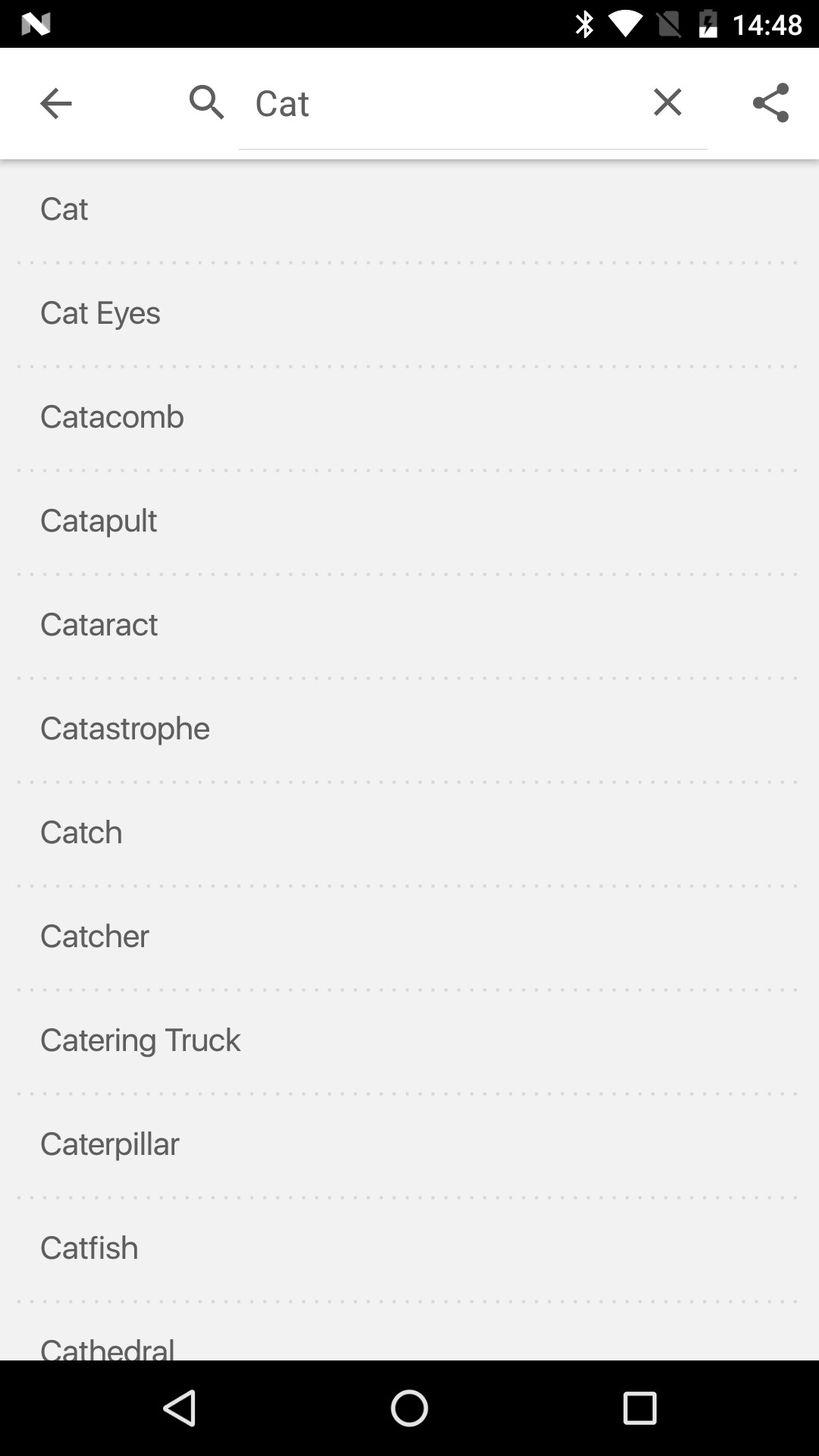A detailed screenshot captured from a cell phone displays a section of the device’s interface. At the top of the screen, various status icons can be seen, including the battery level indicator, the WiFi icon, and the Bluetooth icon. The time is prominently displayed as 14:48. 

Central to the screenshot is a search bar where a user has typed in the word "cat." Below the search bar, a list of autocomplete suggestions is visible, featuring the following terms: cat, cat eyes, catacomb, catapult, cataract, catastrophe, catch, catcher, catering truck, caterpillar, catfish, and cathedral.

Towards the bottom of the screen, a black navigation bar spans the width of the image. On this bar, there are three distinct symbols: a left-pointing arrow, a circle, and a square.

This vertical-oriented image contains no photographic or illustrative elements. Additionally, there are no depictions of people, animals, birds, plants, flowers, trees, buildings, mountains, bridges, automobiles, or motorcycles within this image.